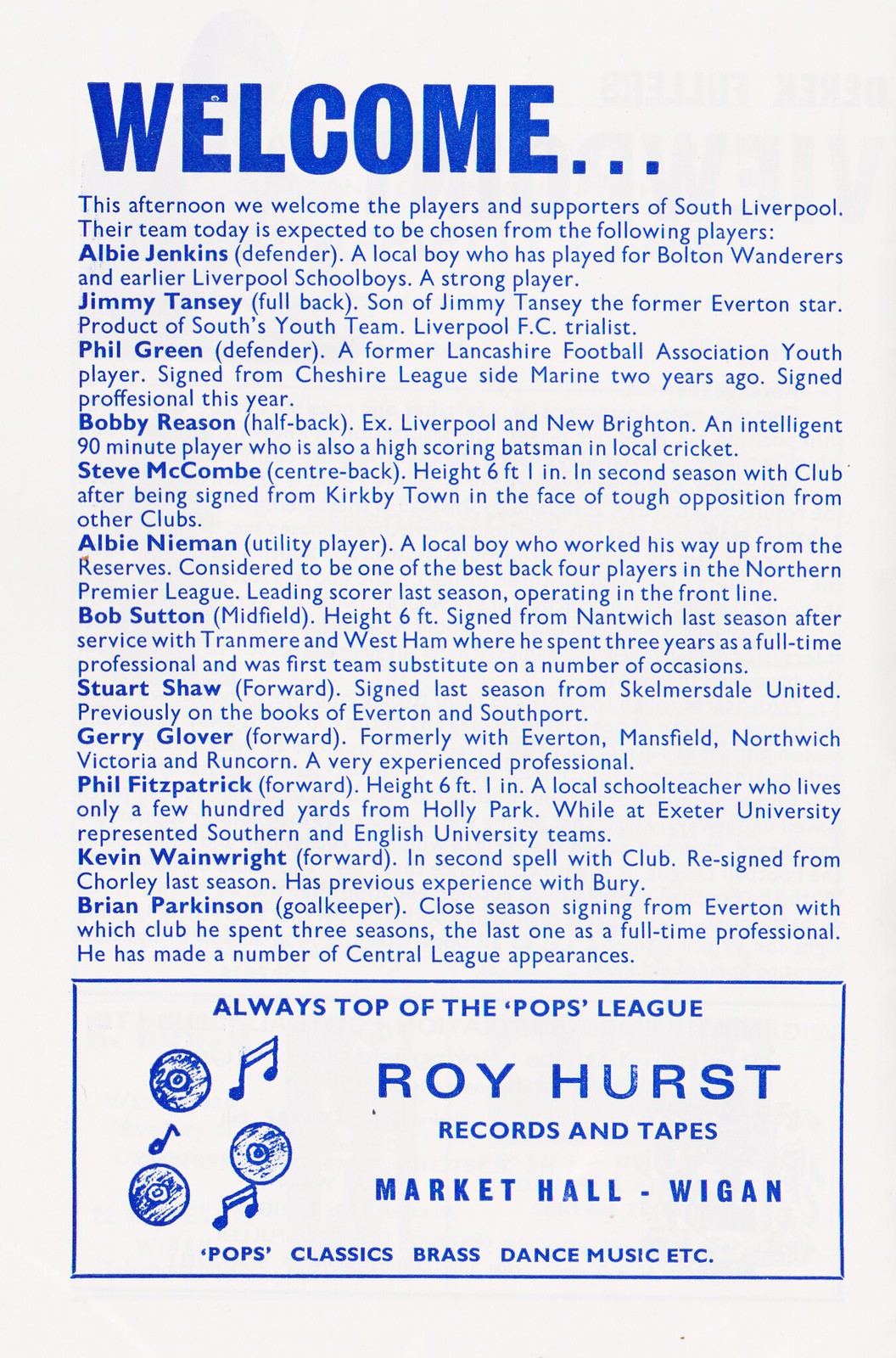The advertisement is a white page with blue lettering prominently featuring the word "WELCOME" in very large letters at the top. Below it, in smaller print, it states, "This afternoon we welcome the players and supporters of South Liverpool. Their team today is expected to be chosen from the following players." Following this introduction is a detailed list of the players, each accompanied by a short biography:

- Albie Jenkins, Defender: A local boy who played for Bolton Wanderers and Liverpool schoolboys, noted for his strength.
- Jimmy Tansley, Fullback: Son of former Everton star Jimmy Tansey, a product of South's youth team, and a Liverpool FC trialist.
- Phil Green, Defender: Former Lynn Shire Football Association youth player, signed from Cheshire League side Marine, and signed as a professional this year.
- Bobby Reason, Halfback: Ex-Liverpool and New Brighton player, an excellent 90-minute player and a high-scoring batsman in local cricket.
- Steve McComb, Centre-back: Standing at 6'1", in his second season with the club after being signed from Kirkby Town amidst tough competition.
- Albie Niemann, Utility Player: A local talent who advanced from the reserves and is considered among the top four players in the Northern Premier League, also last season's leading scorer.
- Bob Sutton, Midfield: 6' tall, signed from Nantwich after serving with Tranmere and West Ham where he was a first team substitute several times.
- Stuart Shaw, Forward: Signed last season from Skelmersdale United, previously with Everton and Southport.
- Jerry Glover, Forward: Formerly with Everton, Mansfield, Norwich, Victoria, and Runcorn, a very experienced professional.
- Phil Fitzpatrick, Forward: 6'1", a local school teacher who lives near Holly Park, represented Southern and English University teams while studying at Exeter University.
- Kevin Weinreit, Forward: In his second spell with the club, re-signed from Chorley, with prior experience at Bury.
- Brian Parkinson, Goalkeeper: Recently signed from Everton after three seasons, with several Central League appearances.

At the bottom of the page, in a boxed section with blue lettering on a white background, the advertisement reads, "Always tops of the Pops League." In large letters, it says "Roy Hurst," followed by smaller letters indicating "Records and Tapes." Below that, in larger letters again, it reads, "Market Hall, Wigan." To the left, there is an image of musical notes, symbolizing CDs or records. The advertisement concludes with the genres "pop, classic, brass, dance, music, etc."